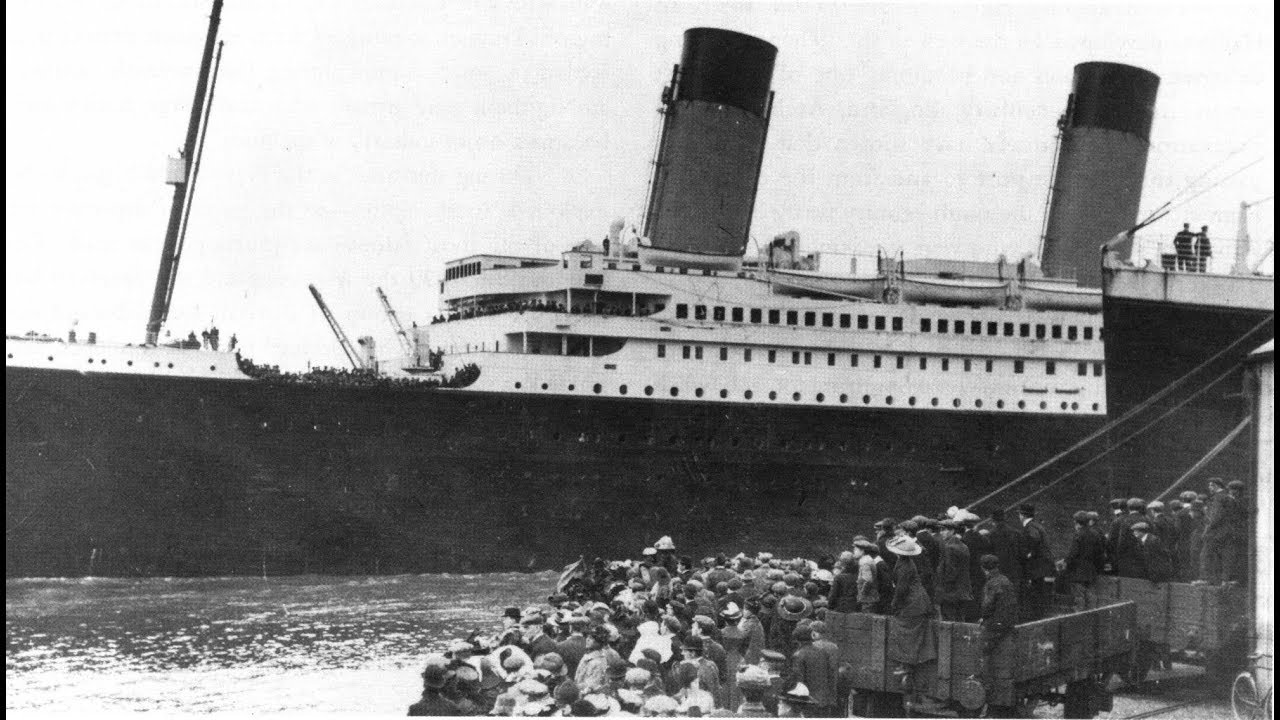This black and white photograph captures a large, vintage steamboat with two prominent steam chimneys at its center, situated on calm waters. The ship, which features a horizontal rectangular section with numerous windows, is adorned with people on its deck, though they appear as indistinct dark figures due to the image's old age. Along the shoreline, a dense crowd of individuals, dressed in what appears to be 18th or early 19th-century attire—women in hats and long skirts and men also in hats—stand either waiting to board or bidding farewell to those departing. The contrast between the ship's black hull and lighter upper structure, though hard to distinguish due to the monochromatic nature of the photo, emphasizes the era's maritime architecture. The overall scene conveys a sense of departure, curiosity, and historical ambience as the populace watches the grand vessel, the focal point of the image, preparing to set sail.